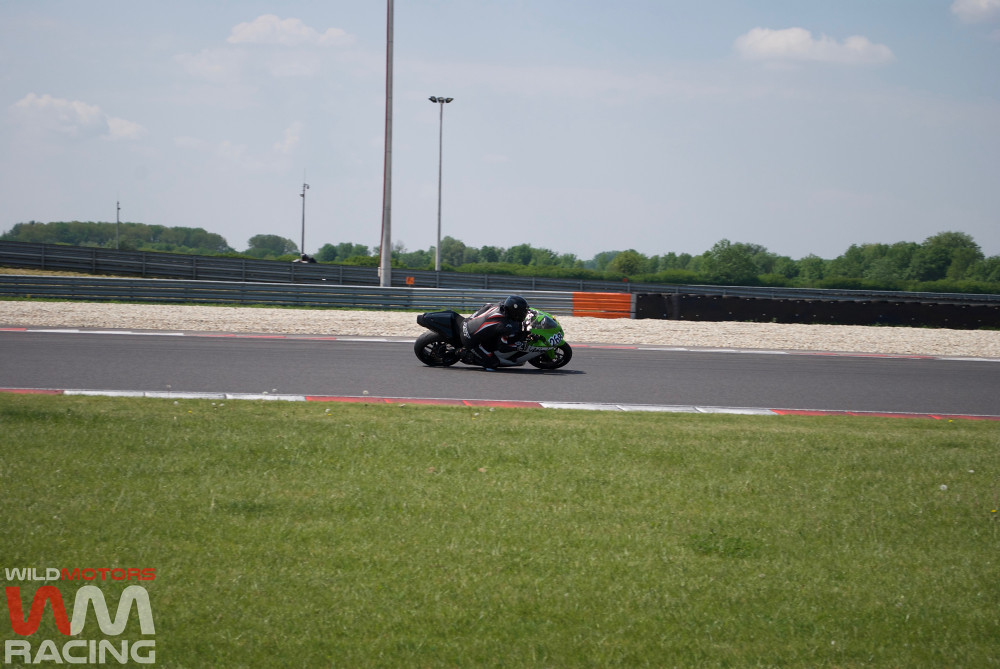This photograph captures an intense moment on a bright, sunny day at a motorcycle racetrack, marked by a nearly cloudless sky. A solo motorcyclist, vividly dressed with a green-fronted motorcycle and a black helmet, is executing a sharp, right-hand turn. The rider is leaning so steeply that his right knee almost grazes the smooth, paved surface of the track, conveying a sense of high-speed agility and calculated risk. The racetrack itself is bordered with red and white striped lines, with a grass field in the foreground and gravel on the far side. Large trees and tall lighting structures stand in the background. Safety barricades, adorned with black barrels or tires, line the track's edge, enhancing the setting's realism. At the bottom left of the image, there is text that reads, "Wild Motions W.M. Racing."